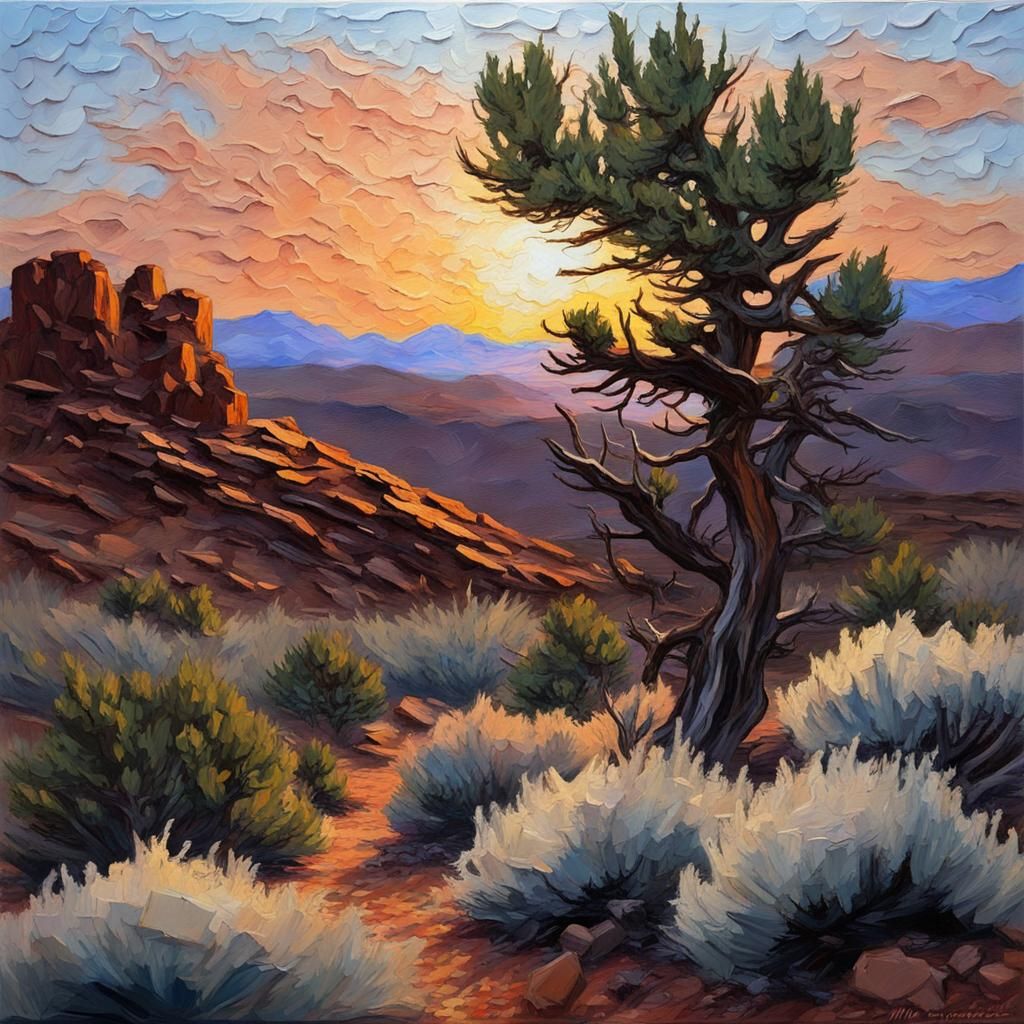The painting depicts a detailed desert landscape, rich with texture, likely created with thick oil paints. Dominating the right side of the image is an old, gnarled tree with textured green leaves and pokey branches reaching towards the sky. At its base, white and green shrubs, tumbleweeds, and dry flowers dot the sandy ground. To the left, a rocky bluff rises prominently, its surface appearing to jut out due to the heavy paint strokes. The background transitions from a vibrant blue sky at the top, through a gradient of orange and yellow hues, resembling a captivating sunset. Further below, the sky turns into shades of purple, accentuating the dusk ambiance. Beyond the bluff, a panorama of higher rocks and mountains in burgundy and blue tones extends into the distance. The setting sun casts its pink and yellow glow, highlighting the rough, wave-like patterns of the painted sky. The scene evokes the rugged beauty of the southwestern desert, with its intricate textures and vivid colors coming together to form a mesmerizing, almost tactile visual experience.